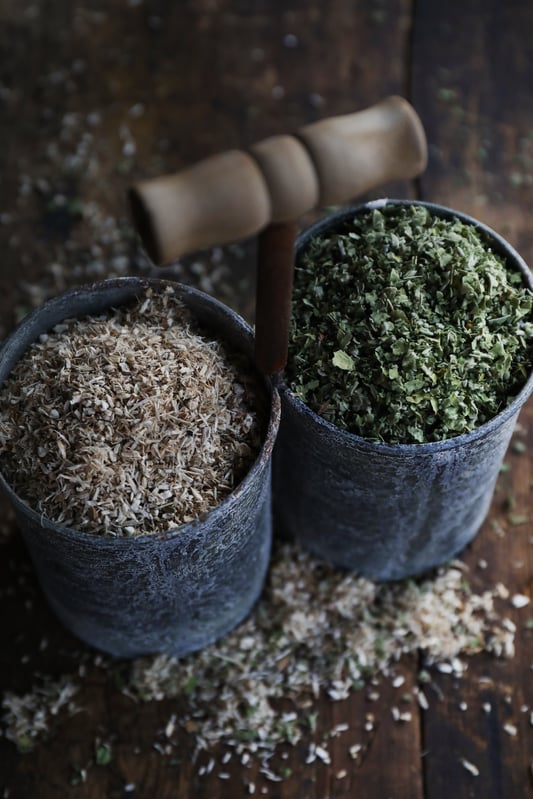This realistic, vertically oriented photograph showcases a pair of unique, deep blue cylindrical containers, possibly handmade, positioned on a brown wooden floor. The containers, which may have once been soup cans now painted denim blue, are connected by a rustic brown wooden handle, allowing them to be carried as a single unit. The left container appears filled with a white, grainy material, potentially sawdust, rice, or another type of grain, some of which has spilled onto the floor. The right container holds a dark green, crumbled herb, possibly dried parsley or oregano, with more of this herb scattered on the floor around and behind the containers. The spilled materials add an organic touch to the scene, with the white grains intermingling with the green fragments on the rich wooden surface. In the background, a lightly colored brown tool, perhaps used for grinding or handling the herbs, quietly completes the rustic and artisanal atmosphere of the photograph.